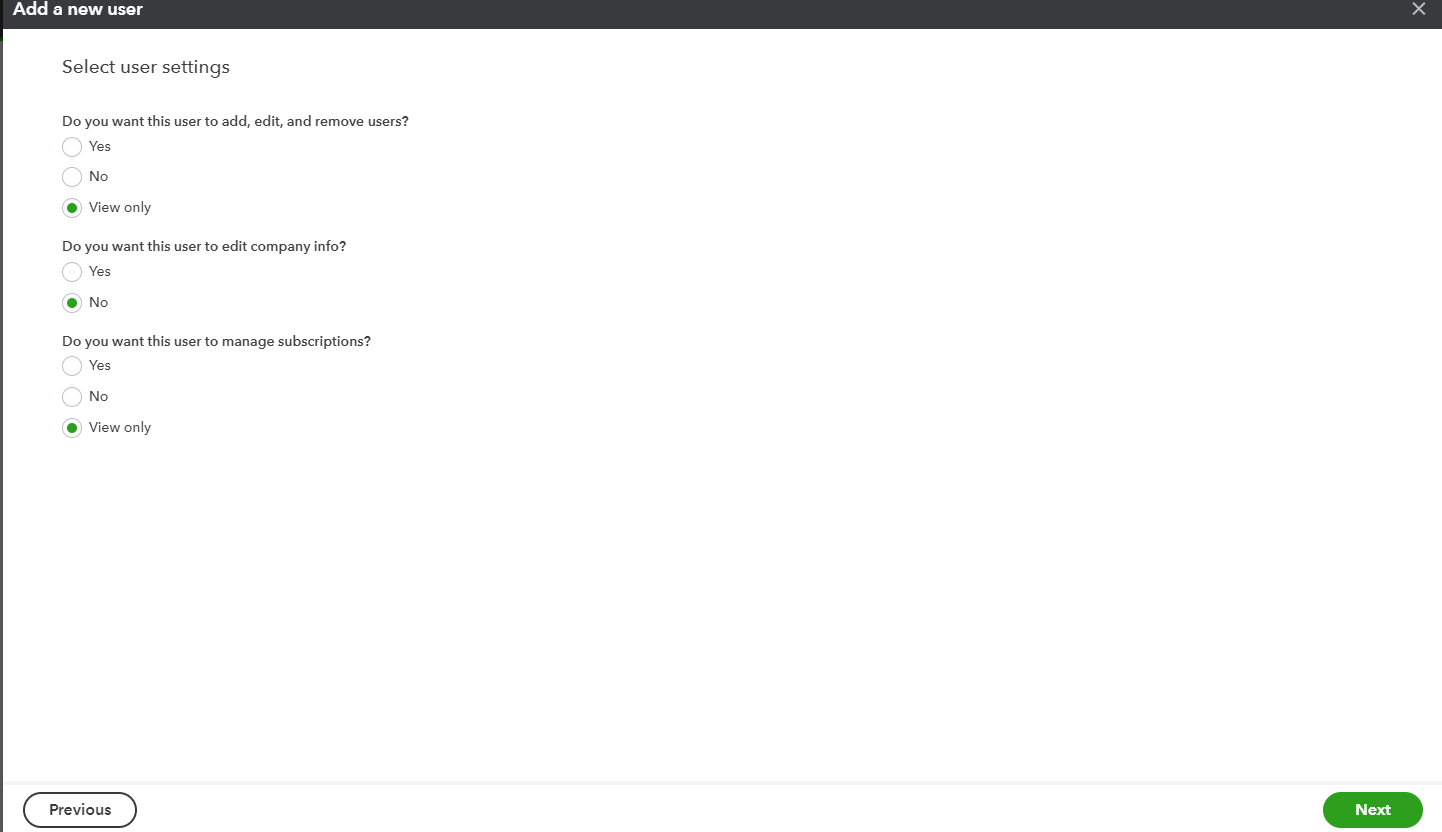The image showcases a straightforward web page with a minimalist design primarily composed of text. At the top of the page, a black navigation bar spans across the screen, featuring white text on the left side that reads "Add New User." On the far right, there is an "X" button for closing the bar.

Below the navigation bar, the rest of the page is purely white with black text, structured as follows:

1. The first line states, "Select User Settings."
2. The next section asks, "Do you want this user to add, edit, and remove users?" followed by checkboxes labeled "Yes," "No," and "View Only." The "View Only" option is selected.
3. The subsequent question is, "Do you want this user to edit company info?" Here, two checkboxes are available, labeled "Yes" and "No," with "No" being checked.
4. The final question posed is, "Do you want this user to manage subscriptions?" with three corresponding checkboxes: "Yes," "No," and "View Only." Similar to the first question, "View Only" is selected.

The page concludes with navigation options at the bottom, allowing the user to go to the "Previous" or "Next" page. This sums up the content and layout of the web page being described.